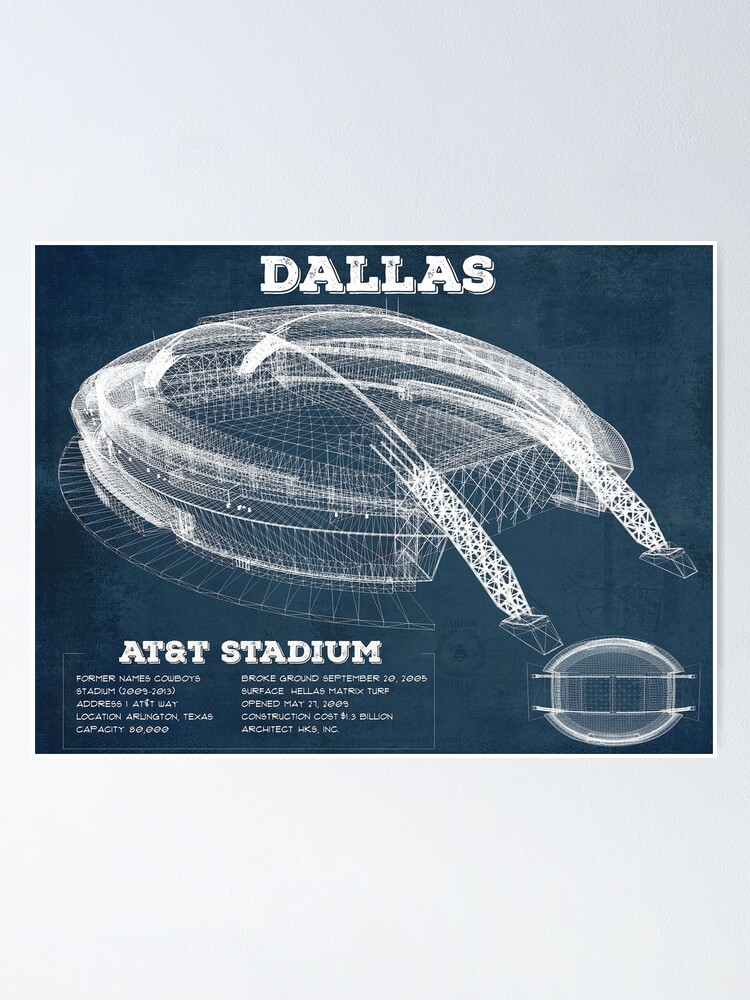This portrait-oriented image showcases a detailed blueprint-style design of the Dallas AT&T Stadium against a grayish off-white background. At the top, the word "DALLAS" is prominently displayed in all caps in white. Central to the image is a dark blue rectangle bordered in white, within which AT&T Stadium is written at the bottom. In the lower left corner, additional text details include the stadium’s former names, Cowboys Stadium (2009-2013), its address at 1 AT&T Way, Arlington, Texas, and a seating capacity of 80,000. Adjacent to these, the right column lists key dates and attributes: the groundbreaking on September 20, 2005, surface type (Hellas Matrix Turf), opening date (May 21, 2009), construction cost ($1.3 billion), and architect (HKS Inc.). The lower right corner features a white overhead drawing of the stadium. Centrally, a detailed white rendering of the stadium from an overhead and partially angled perspective dominates the image, providing intricate architectural details of the structure.